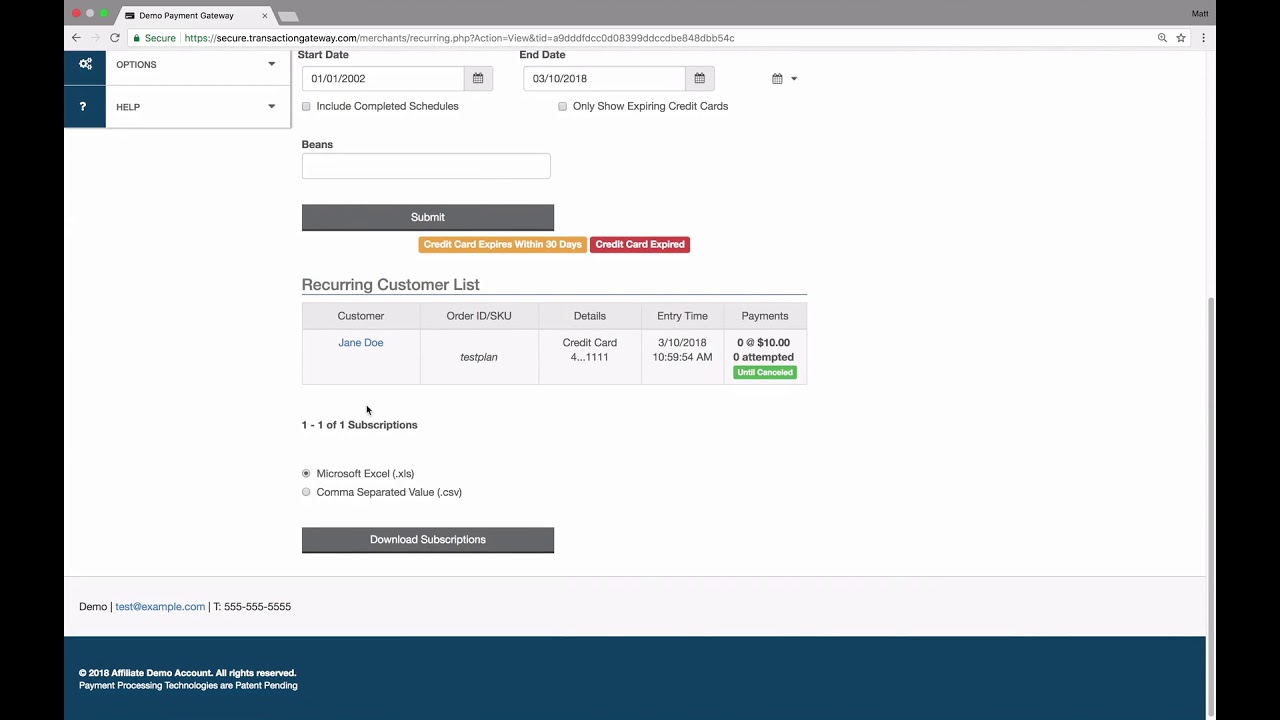The image displays a web page of a payment gateway, specifically titled "Demo Payment Gateway." The URL appears to be "secure.transactiongateway.com/merchant/recurring/[additional characters]," indicating a secure transaction platform. The user seems to be accessing the page on an Apple desktop, as indicated by the characteristic red, gray, and green buttons located in the top left corner of the screen.

In the main section of the page, two tabs are visible: an "Options" tab with a dropdown menu, denoted by a down arrow, and a "Help" tab that also features a dropdown arrow for additional options. 

The form on the central portion of the page includes an entry box for specifying a start date and an end date, which are populated as "January 1, 2002" and "March 10, 2018," respectively. Below these date fields, there is an entry box labeled "Beans." Adjacent to these fields is a gray "Submit" button.

Further down, the page displays a section titled "Recurring Customer Lists," showing details of a customer named Jane Doe. Included in this section are specifics of a credit card transaction: the entry time marked as "March 10, 2018," and a payment amount of "$10." At the bottom of the page, there is another gray button labeled "Download Subscriptions."